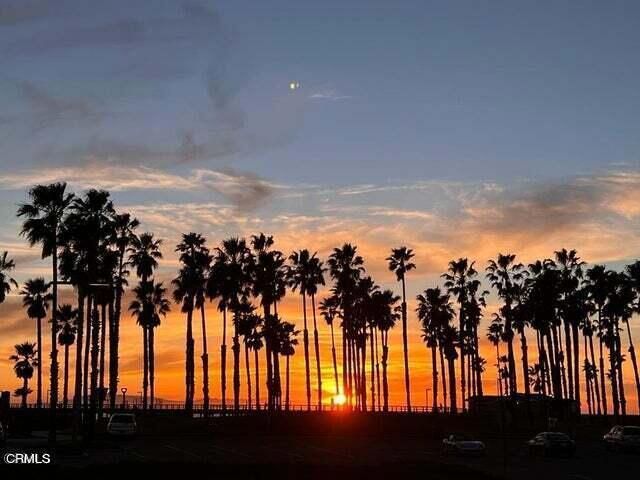In this outdoor photograph taken at dusk, the sky is a captivating blend of colors transitioning from blue at the top to shades of pink, orange, and yellow closer to the ground. White, purple, gray, and orange clouds scatter across the sky. The sun, appearing yellowish, is setting near the horizon in the center of the image, giving a warm glow to the scene. A row of palm trees stretches across the width of the photo, casting dark outlines against the colorful sky. In the foreground, there's a dimly lit parking lot with a handful of parked cars, including a notable truck, and a railing suggesting a sidewalk. Streetlights add subtle structure to the scene. Text reading "CRMLHS" is visible in white in the bottom left corner.